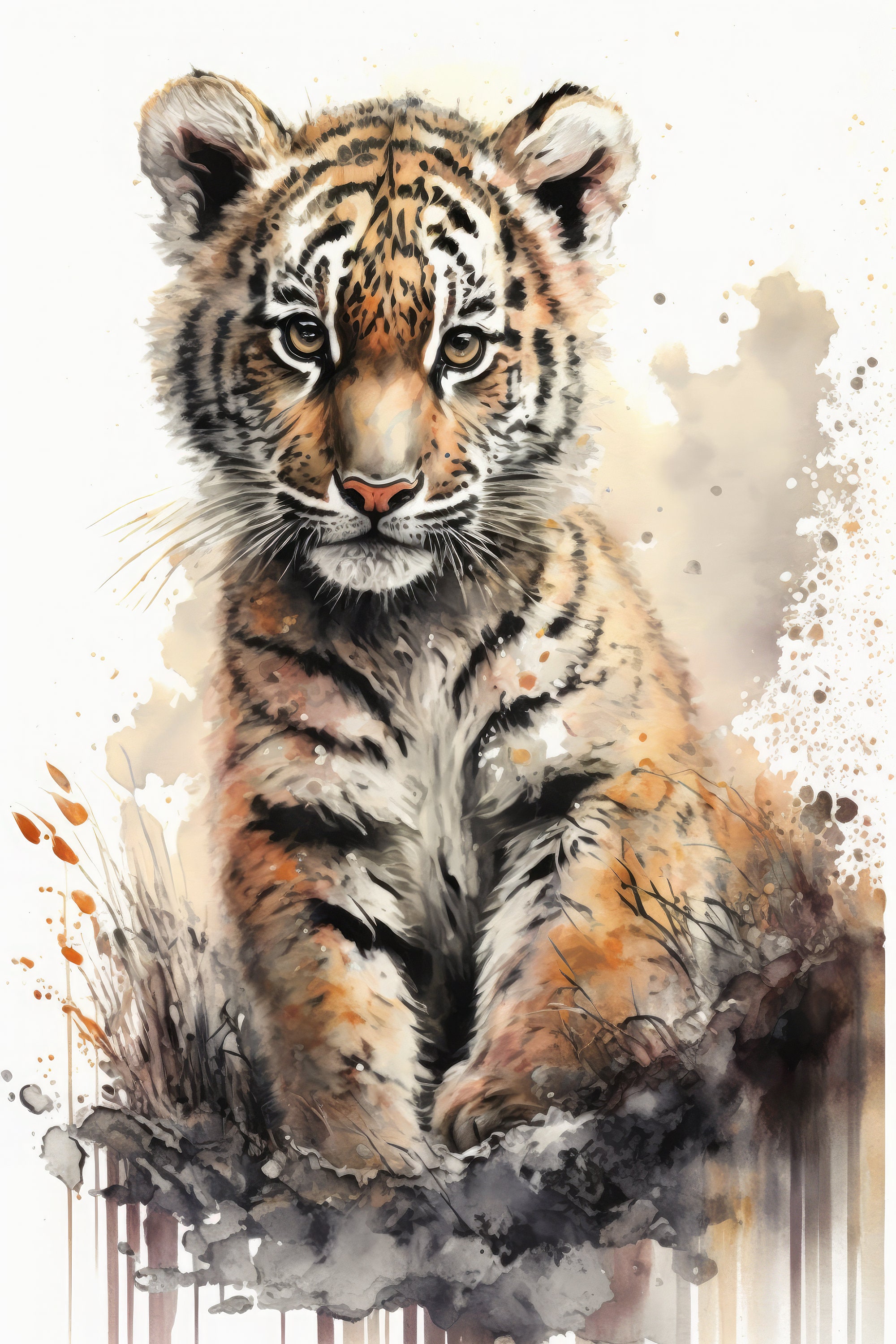The image is a detailed watercolor illustration of a young tiger cub, sitting on the ground with its two front paws positioned in front of it. The tiger cub gazes thoughtfully or mournfully straight ahead at the viewer, with striking light brown, amber-like eyes and black pupils. Its fur showcases the typical tiger pattern with shades of orange, black stripes, muted dull brown, white, and cream. The illustration captures the cub with fine details, making it easy to distinguish individual patches of hair. The nose of the cub is distinctly orange.

The painting transitions into a more abstract style towards the bottom, where colors begin to blend together more fluidly. Below and around the tiger, the background features splatters and splotches of watercolor, in shades of beige, taupe, and dull orange, creating a sense of a wet, spontaneous painting process. These splatter marks also appear beneath the tiger's paws and extend into the backdrop, suggesting an outdoor setting. The overall composition merges both realistic and impressionistic elements, illustrating a young tiger cub with a serious demeanor against an artful, loosely painted background.